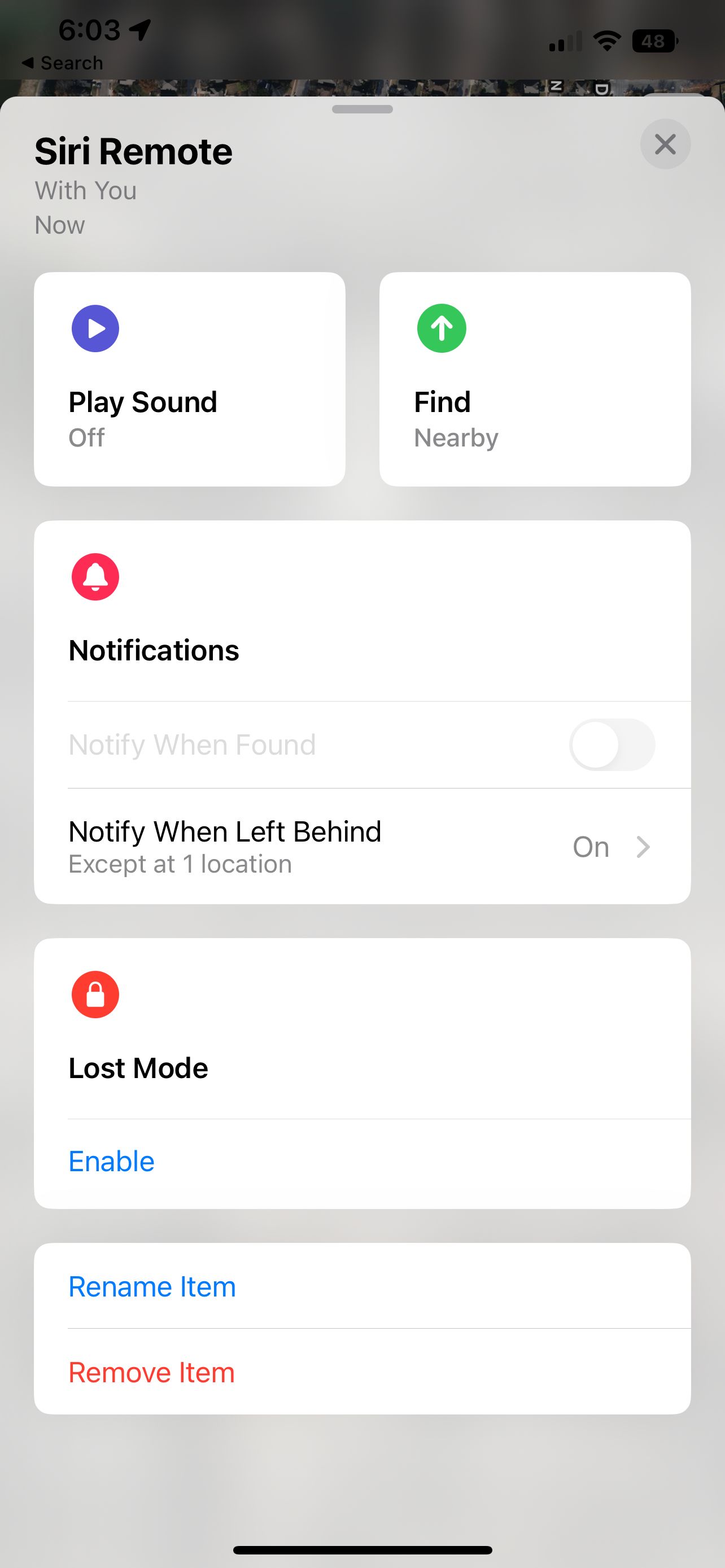The image appears to be a screenshot taken from a cell phone, showcasing a user interface with various options and controls. The top part of the image is obscured by a darker gray shadow, and a faint battery icon is barely visible in the top right corner. Below this, there is a long gray rectangular section.

At the beginning of this section, "Siri Remote" is written in black text. Beneath that, there is a horizontal lineup of smaller gray squares with different functionalities:

- The first square features a white interior with the words "Play Sound" inside it, and above this is a purple circle with an arrow icon.
- The second square reads "Find" in black text, with a green circle and an arrow pointing upwards above it, and the word "Nearby" located underneath.

Following these are larger sections with additional options:

- A larger square contains a red circle with a bell icon, labeled "Notifications," with the option "Notify When Left Behind Except At One Location" displayed beneath it. This option is currently enabled.
- Another larger square features a red circle with a white lock icon, labeled "Lost Mode," with the word "Enable" in blue text below it.

Finally, towards the bottom:

- There is a blue text option that says "Rename Item."
- Below it, a faint gray line separates this from another red text option, "Remove Item."
- At the very bottom-center of the image, a horizontal black line approximately four inches long is present, possibly part of the interface design.

This detailed description covers various elements and options available in the screenshot, providing a comprehensive view of the image's content.